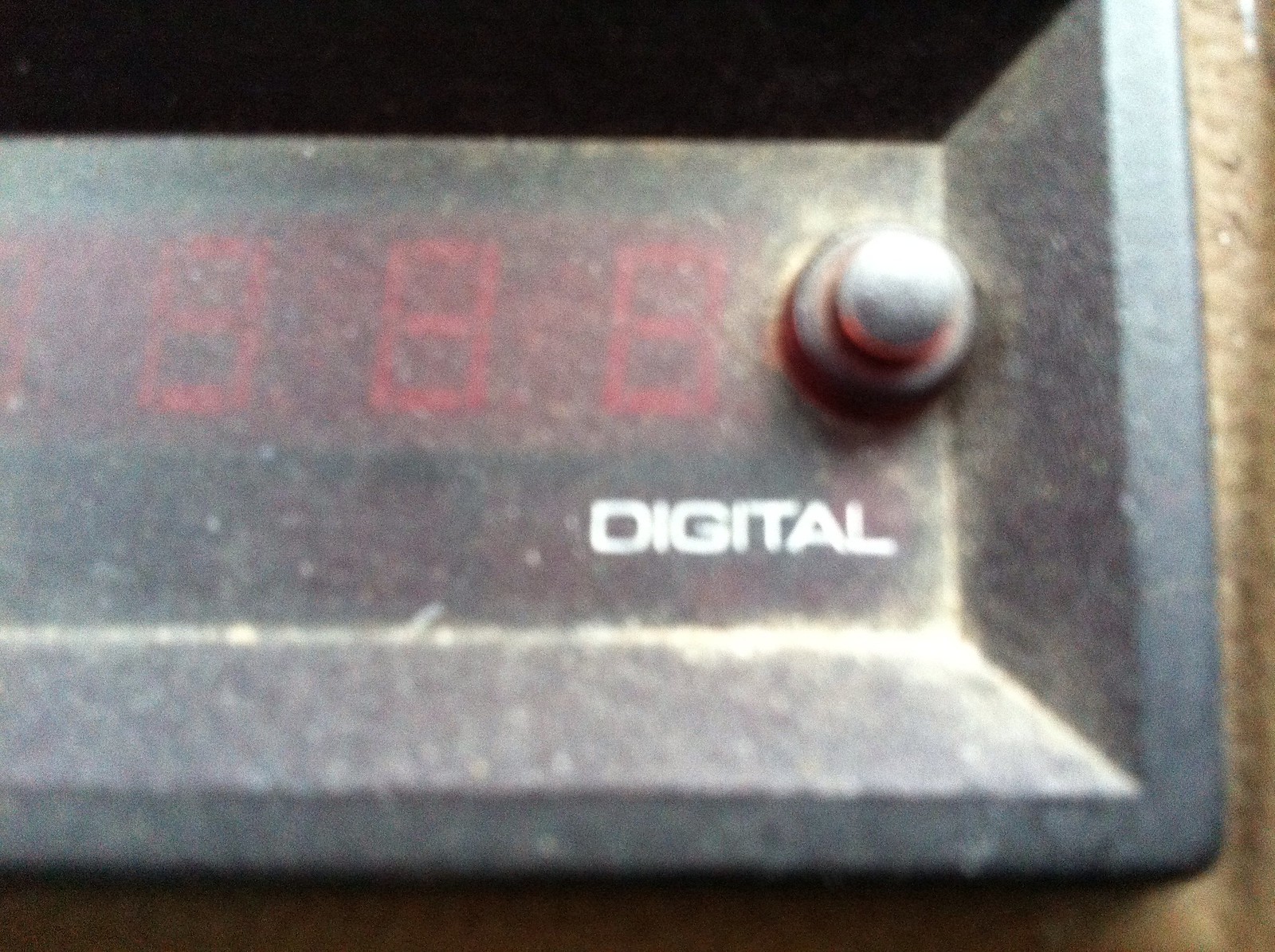This photograph captures an extreme close-up of an electronic device, likely a clock. The background is a muted brown, providing a neutral backdrop that accentuates the device's features. At the center, a white rectangular panel is bordered by a black frame that extends downwards into a concave structure, made of sleek black plastic. Dominating the panel is a prominent digital display, where vivid red numbers are clearly visible. To the right, a small, metallic silver button stands out, adding a tactile element to the device. The word "Digital" is printed in crisp white lettering, reinforcing the device's modern functionality. The meticulous detailing and structured composition yield a compelling visual narrative of contemporary technology.